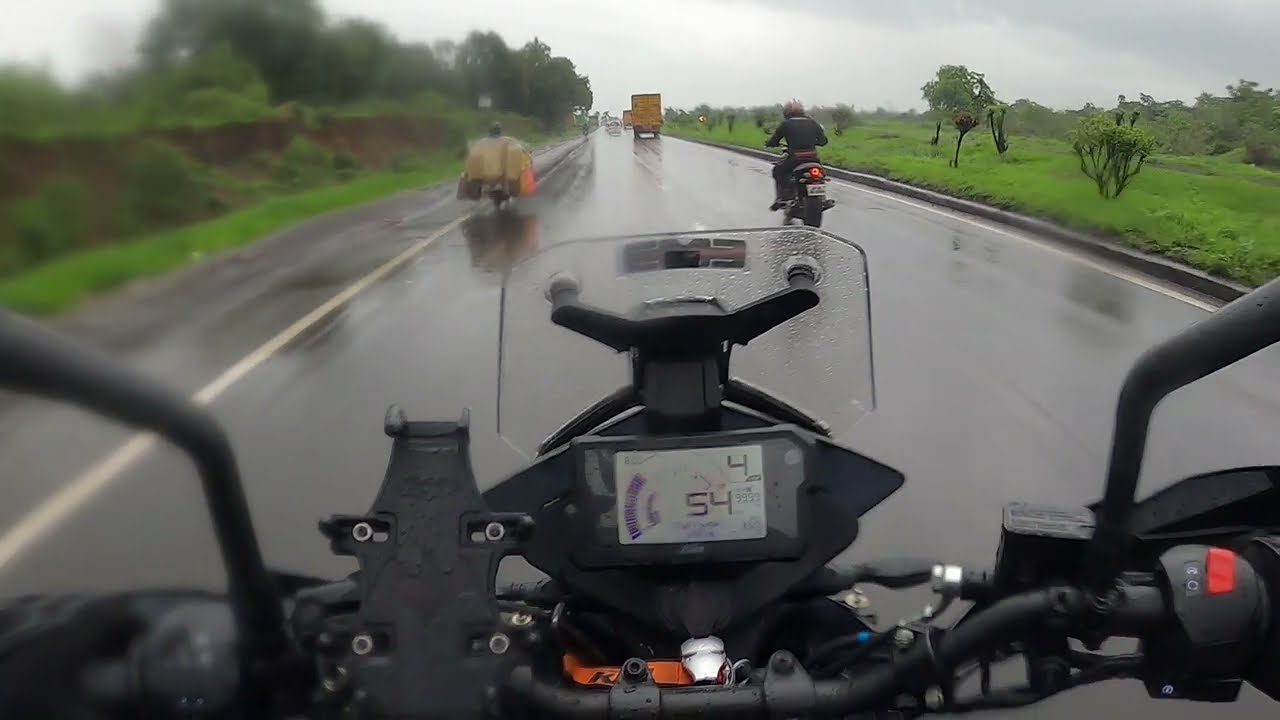The photograph captures the point of view of someone riding a motorcycle on a rainy day. In the center of the image is the motorcycle's speedometer, mounted on the center console, displaying a speed of 54 miles per hour. The windscreen, positioned above the speedometer, is speckled with raindrops. The road ahead is a dark gray asphalt strip, marked by a white dotted line in the middle, flanked by solid white lines on the edges. To the right of the road, there is a curb, behind which lies a mostly flat green area populated with small trees and patches of grass. On the left, a small hill is visible, its slope adorned with patches of bare dirt, grass, and more green trees. The road is a one-way route, extending forward, with the motorcyclist potentially accompanied by other vehicles, including scooters, Vespas, and possibly a trailer truck. The scene is framed by the misty, rain-soaked atmosphere, adding a sense of motion and weather conditions to the journey.